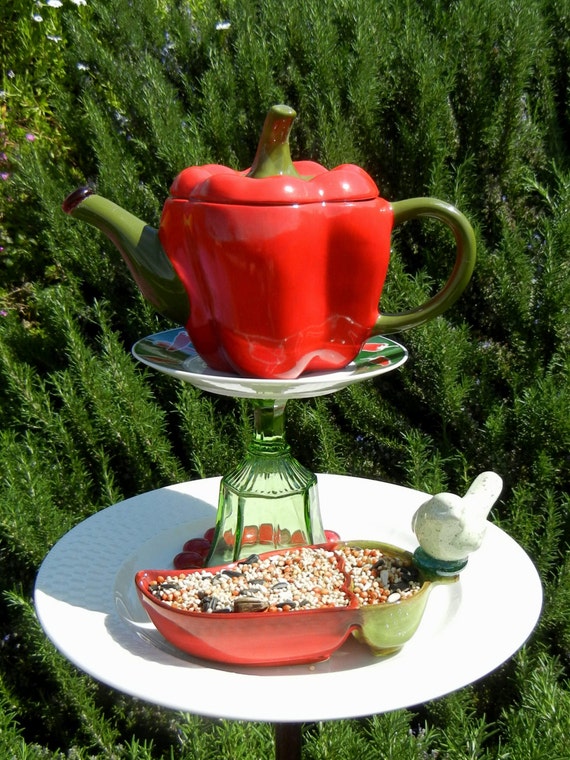The photograph depicts a whimsical arrangement set against a backdrop of dense, dark green foliage with long, spiky leaves. Centrally featured is a stack comprising several items, each artfully placed atop the other. At the base is a white porcelain plate, which appears elevated above the ground, suggesting it might be on a stand. Upon this plate sits an upside-down, light green glass goblet. Balancing on the base of the inverted goblet is another small, white saucer.

At the top of the stack rests a unique teapot designed to resemble a red bell pepper, complete with a green stem, handle, and spout. The red pepper body of the teapot is vibrant, adding a pop of color to the composition. Within the setup, another element resembling a bowl shaped like a pepper, possibly meant to evoke the appearance of a duck, is filled with small white and red pebbles. This imaginative arrangement of everyday objects contrasts sharply with the natural edginess of the background vegetation, resulting in a whimsical yet detailed scene.